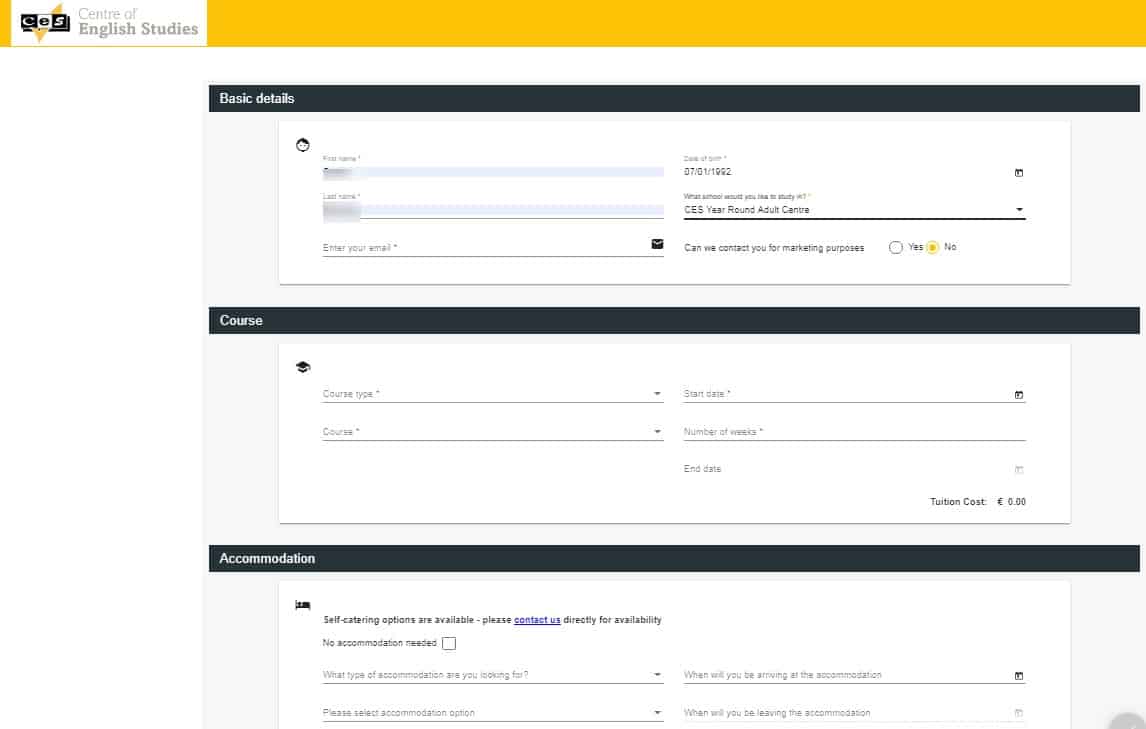This image depicts a webpage from the "Center of English Studies." The user interface is laid out with a black and white themed image on the left, highlighted by an orange border stripe. This image and border sit atop an orange bar that spans horizontally across the page. 

Below the image area, there's a black bar labeled "Basic Details," where users are prompted to enter their first name, last name, email address, and the current date. There's also a small, pre-filled text that reads "year-round adult center." Another section asks, "Can we contact you for marketing?" to which the user has selected "No." 

A form area for the course details is next, where users can specify the type of course they wish to enroll in. This section also contains a field that calculates the tuition cost, positioned towards the lower right of the interface.

Moving on to the next section, labeled "Accommodation," it mentions that self-catering options are available, prompting users to contact them for availability, with a clickable “Contact Us” link in blue. Users can also specify the type of accommodation they need in this area. The text is small but legible, although part of the page appears to be cut off, indicating that further form details are available by scrolling or navigating further. The layout and font are designed to be clear and user-friendly, enabling users to fill in the required information with ease.